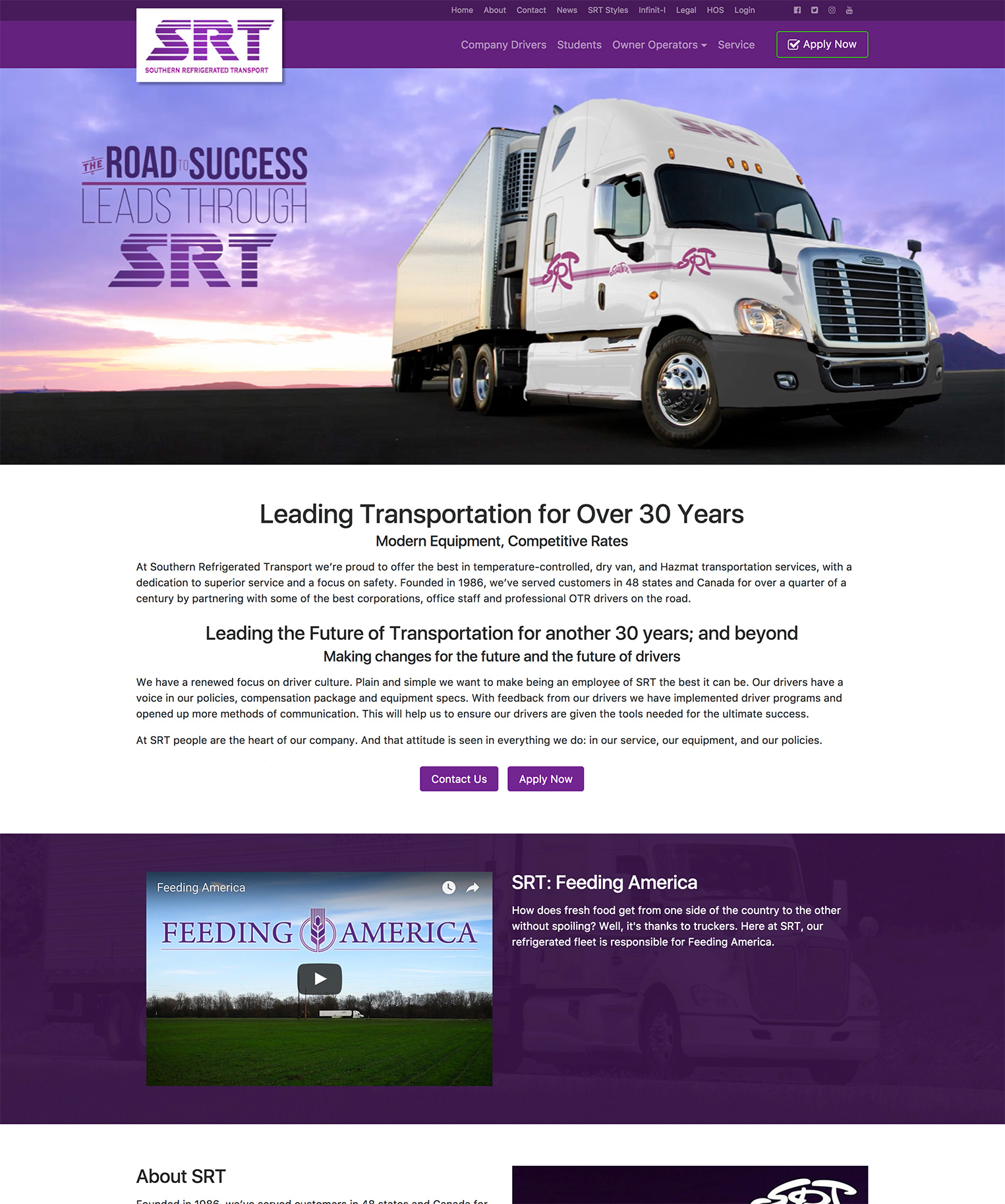The image depicts a recruitment advertisement for Southern Refrigerated Transport (SRT), featuring a prominently purple-themed landing page. At the top, a narrow, dark purple band includes menu options such as Home, About, Contact, News, SRT Styles, Infinite-I, Legal, HOS, HDS, and Login. Below this, a slightly lighter purple section provides quick links for Company Drivers, Students, Owner Operators, Service, and Apply Now.

The central focus of the page is a dramatic photograph of a semi-truck hauling a refrigerated trailer, captured at dusk. The scene presents the truck emerging from the center of the image, moving towards the lower right-hand corner, against a backdrop of a twilight sky tinged with deep blues and purples. Overlaying this image, the motivational text reads, "The Road to Success Leads Through SRT," followed by a descriptive blurb about SRT’s industry leadership: "Leading transportation for over 30 years, modern equipment, competitive rates."

Additional promotional text reinforces the company's future-oriented vision: "Leading the future of transportation for another 30 years and beyond. Making changes for the future and the future of drivers." Prominently featured calls-to-action like "Contact Us" and "Apply Now" encourage prospective drivers to engage further.

Towards the bottom of the image, a very dark purple box highlights SRT’s mission with text that reads: "SRT, Feeding America. How does fresh food get from one side of the country to the other without spoiling? Well, it's thanks to truckers. Here at SRT, our refrigerated fleet is responsible for feeding America." A video titled "Feeding America" can be played to learn more about their operations.

Lastly, the webpage extends to include an "About SRT" section, juxtaposing descriptive text on the left with a blacked-out image area on the right, though both are slightly cropped, limiting full visibility.